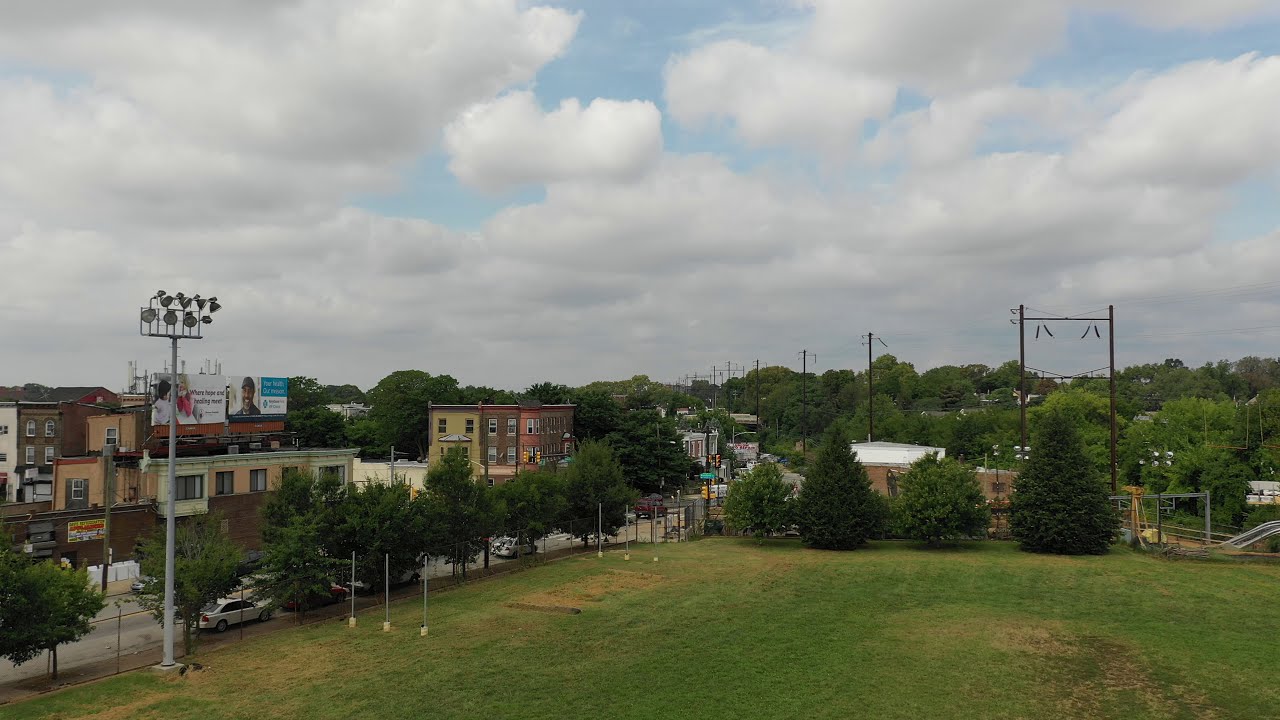This high-angle, daytime photograph showcases a small town’s neighborhood with intricate details divided between the sky and the landscape below. The upper portion of the image is filled with large, white, fluffy clouds, tinged with light gray at their undersides, floating low enough to feel almost touchable atop a tall tree. Against this backdrop, blue skies peek through, creating a picturesque scene.

The lower half of the photograph reveals a spacious, empty, grassy field, likely a park, bordered by a chain link fence adorned with trees. To the left of the field stands a tall spotlight, perfect for illuminating nighttime soccer games. Surrounding the park are a mix of tall, brown buildings, several cars, and a network of power lines crisscrossing through the scene. The road glimpsed in the background stretches deep into the distance, emphasizing the town’s layout. This digital photograph, possibly captured from a drone, incorporates a rich palette of greens, whites, yellows, reds, browns, blacks, blues, and hints of pink, capturing the vibrant essence of this quaint small-town neighborhood.